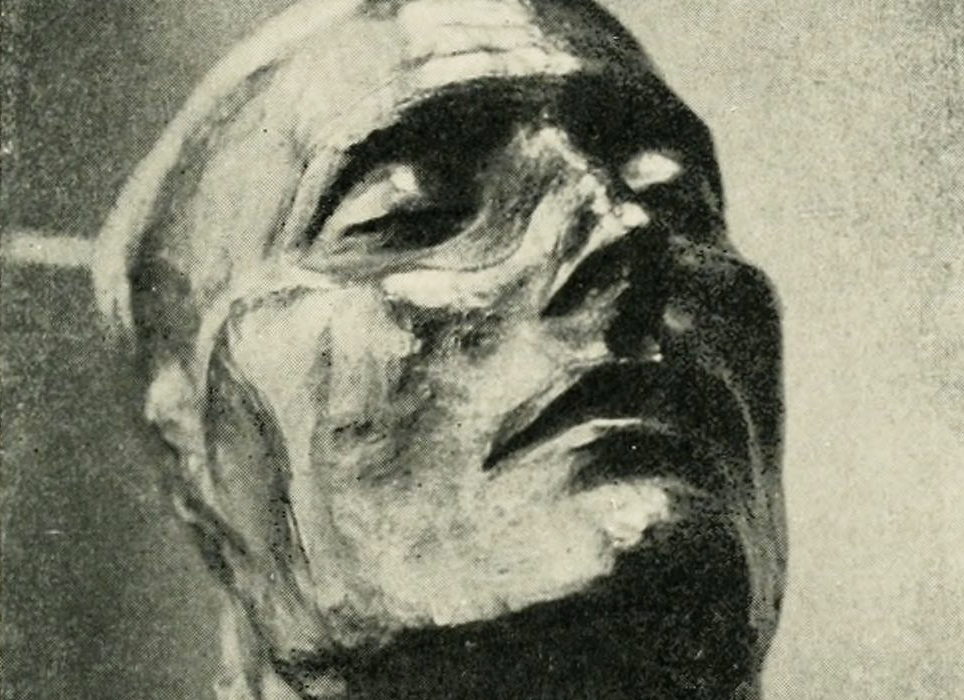The image depicts a highly detailed, black and white charcoal drawing of a lean male face, taking up almost the entire frame. The man's eyes are closed, giving the appearance of either serene contemplation or rest. His head is tilted back, looking upwards, with closed lips and a pronounced, pointy chin. The man's high cheekbones are sharply defined with shadowing accentuating his facial contours, particularly around the bridge of his nose and the cheeks. The ears are not detailed, and the hair is either very short or not present. The background features a grainy, gradient texture transitioning from dark gray to light gray, enhancing the stark contrast of the face. Slight light seems to emanate from the left side, casting subtle highlights on the left bridge of the nose and the eyelids, contributing to the dramatic effect of the composition. The drawing combines areas of deep shadow, particularly beneath the chin, with prominent outlines of facial features, creating a striking and enigmatic portrayal.